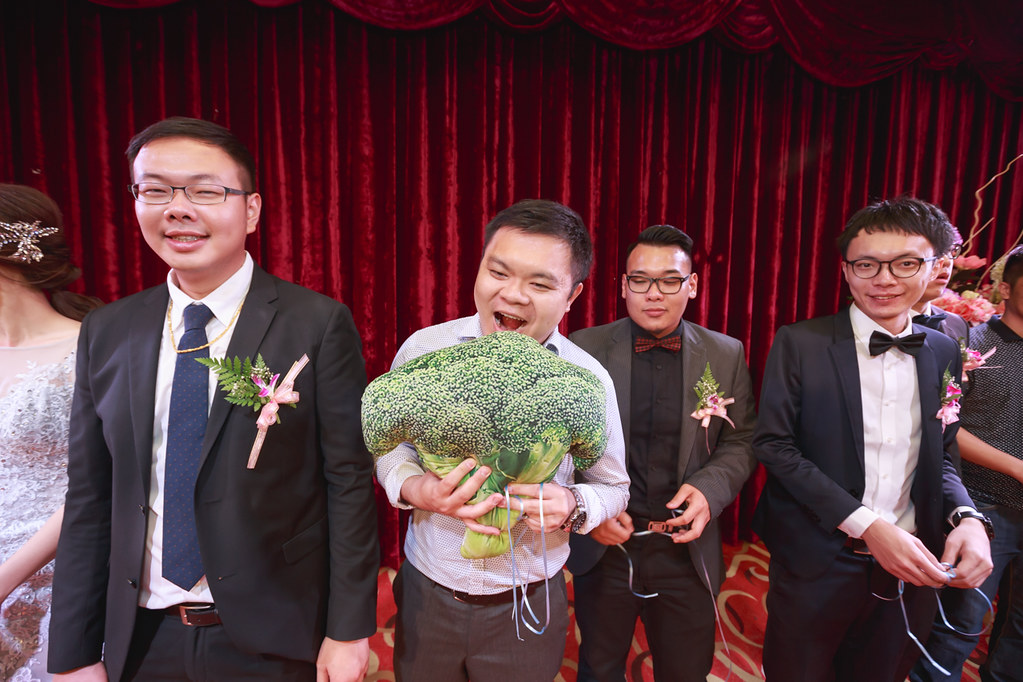In this color photo, a group of Asian individuals is standing mostly in a straight line before a deep red, velvety curtain, suggesting a ceremonial or stage setting. The group includes four men and a partially visible woman on the left. The woman, dressed in white with a hair clip, has her back to the camera. 

The first man on the left is smiling broadly, sporting glasses, a blue tie, a white collared shirt, a blazer, and a corsage with a pink ribbon on his lapel. Beside him, a man is holding an oversized, realistic-looking broccoli floret with both hands, his mouth open as if pretending to take a bite. He is not wearing a suit jacket but is dressed in gray dress pants, a button-up shirt, and is also holding a blue string around his left hand. 

Next in line is a bespectacled man wearing a red and black bow tie, a gray blazer, and a similar corsage. Following him is another man in glasses, black hair, a black bow tie, and a tuxedo, also adorned with the same style of corsage. Two more people are partially visible behind him, though their details are unclear.

The men appear well-dressed, mostly in suits with flower corsages, and each one is holding a ribbon. The infusion of whimsical elements like the giant broccoli adds an intriguing touch to the formal attire and setting.